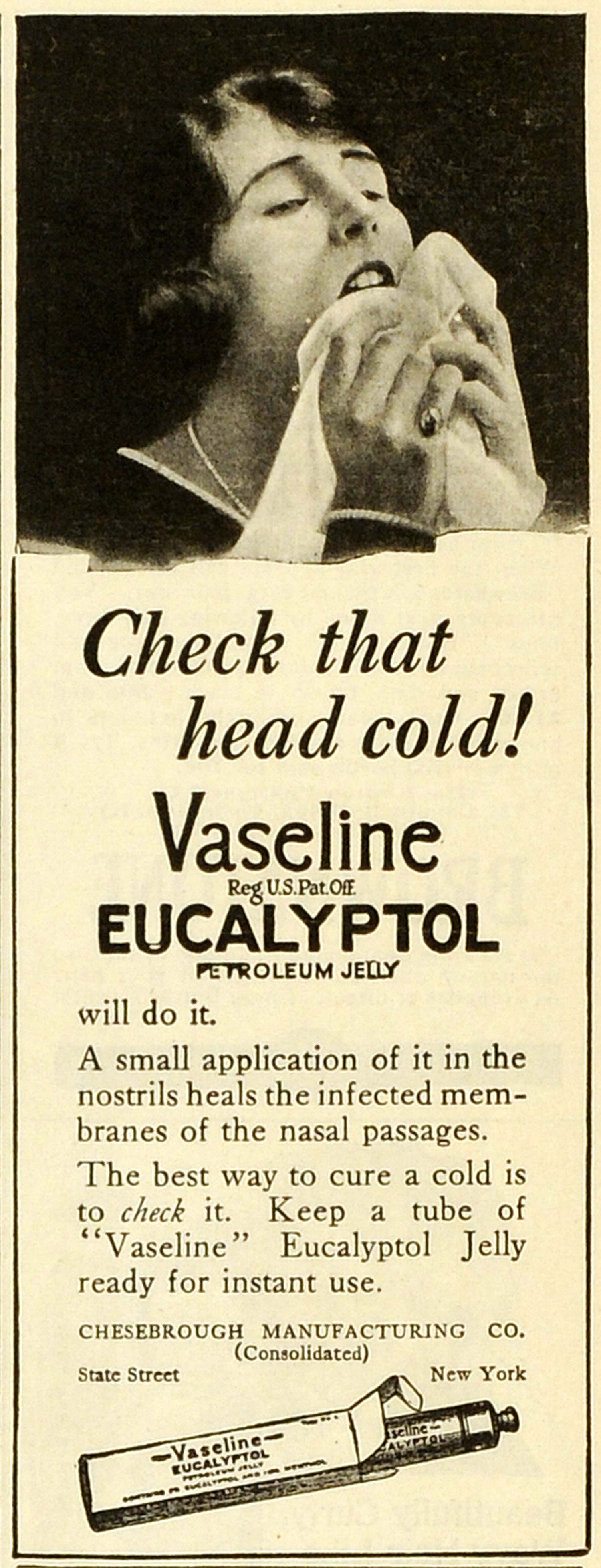The advertisement, dating back to the 1920s or 1930s, is a rectangular print showcasing a black and white image of a woman at the top. Her eyes are closed, her head is leaning back, and her mouth is slightly open with a cloth resting on her bottom lip. She wears a white necklace, which stands out against the grayscale image.

Beneath the image, on a beige background, bold black text reads: "Check that head cold." Intriguingly, the exclamation point is replaced with the word "Vaseline." Below that, the text "REG. U. S. PAT. OFF." appears, followed by a pitch for "Vaseline Eucalyptol Petroleum Jelly," which claims to heal the infected membranes of the nasal passages with a small application in the nostril. The advertisement emphasizes the importance of addressing a cold promptly and suggests keeping a tube of Vaseline Eucalyptol Jelly ready for instant use.